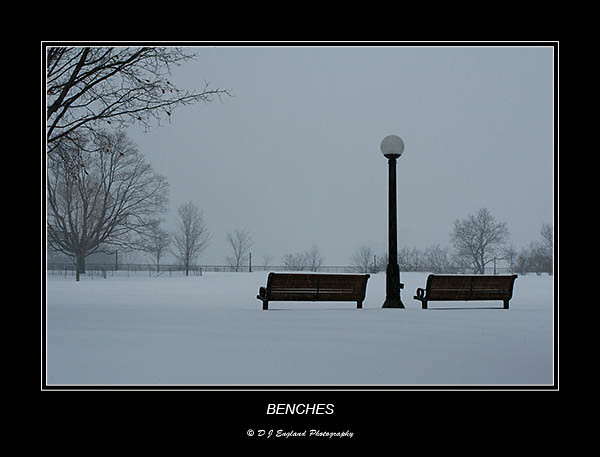The black-and-white photograph, titled "Benches" in white text along the bottom border, credits DJ England Photography. The image is framed by a black border which also includes the signature "DJ England" in cursive. Central to the scene are two wooden benches seen from behind, placed in the middle of a snowy field. A black lamppost with a round white globe light stands between the benches. The background features a line of leafless trees, indicative of winter, with some stretching tall while others are slightly shorter, creating a gradient of height towards the center. The sky appears hazy, alluding to a recent snowstorm, and a fence line recedes into the distance, leading the eye towards the center of the image. The overall composition evokes a serene, quiet winter landscape.